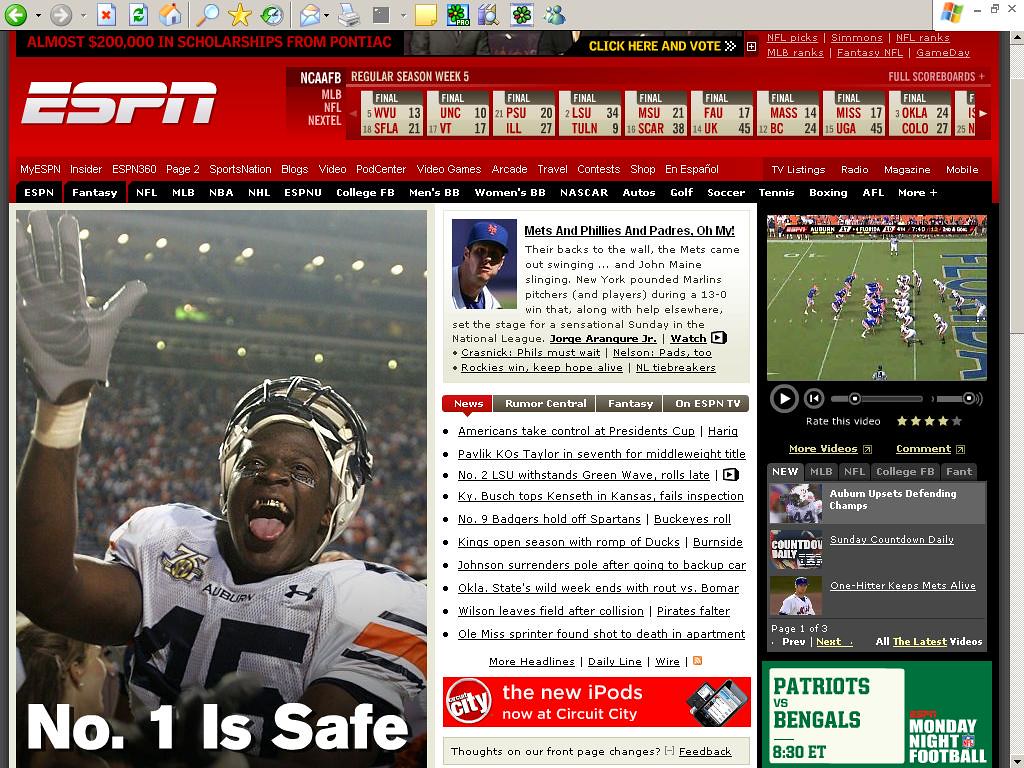The screenshot features a vintage ESPN website from what appears to be the late 1990s or early 2000s, showcasing the web design and sports content typical of that era. Dominating the page is a headline proclaiming "The Number One is Safe," accompanied by an image of an elated football player whose team is indeterminate. 

Above the headline, there are navigation links for various sports including MLB, NFL, and Nextel Cup Series, as well as an option to view full scoreboards, suggesting it's around week five of their seasons. The site's header includes a plethora of options such as My ESPN Insider, ESPN 360, Page Two, Sports Nation, Blogs, Video Pod Center, Video Games, Arcade, Travel, Contests, Shop, and Español, offering a broad array of content beyond just sports news.

The main articles highlighted on the page include one with the title "Mets and Phillies and Padres, Oh My," likely discussing a significant development in baseball. Beneath these articles lies a news section focusing on various topics, which appear to predominantly feature college sports updates. This densely packed webpage reflects the multi-sport focus and broad appeal that characterized ESPN's early digital presence.